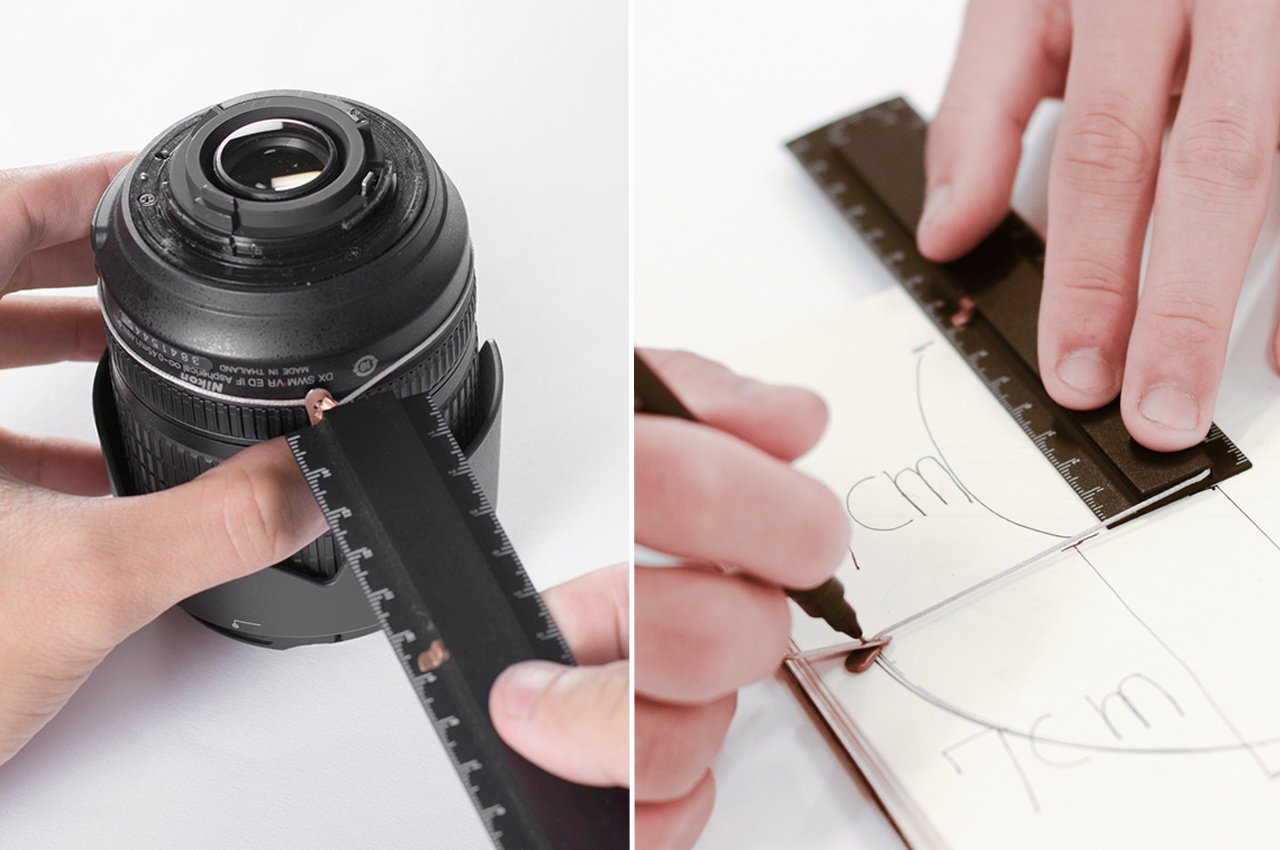The detailed image consists of two vertically rectangular, professionally staged, full-color photographs side-by-side, separated by a thin white line. The overall composition is square and was shot indoors under artificial lighting. 

On the left side of the image, a pair of Caucasian hands is visible, handling a black Nikon camera lens. The lens features subtle white accents and a distinguishable swivel area, with a hint of glass visible at the top. The person is holding the lens with their left hand and a black ruler marked with white measurement lines in their right hand, aligning it to the lens. The setting appears staged against a plain white background.

On the right side, the same hands are shown using the ruler and a pen to draw on a white piece of paper. The fingers, cropped close to the nails, precisely measure and sketch, including straight and curved lines. Clearly visible are the numbers "7 CM" and various curves, hinting at mathematical or technical drawings correlating with the measurements taken from the camera lens. This part of the image also features a white background, maintaining a clean and minimalistic aesthetic.